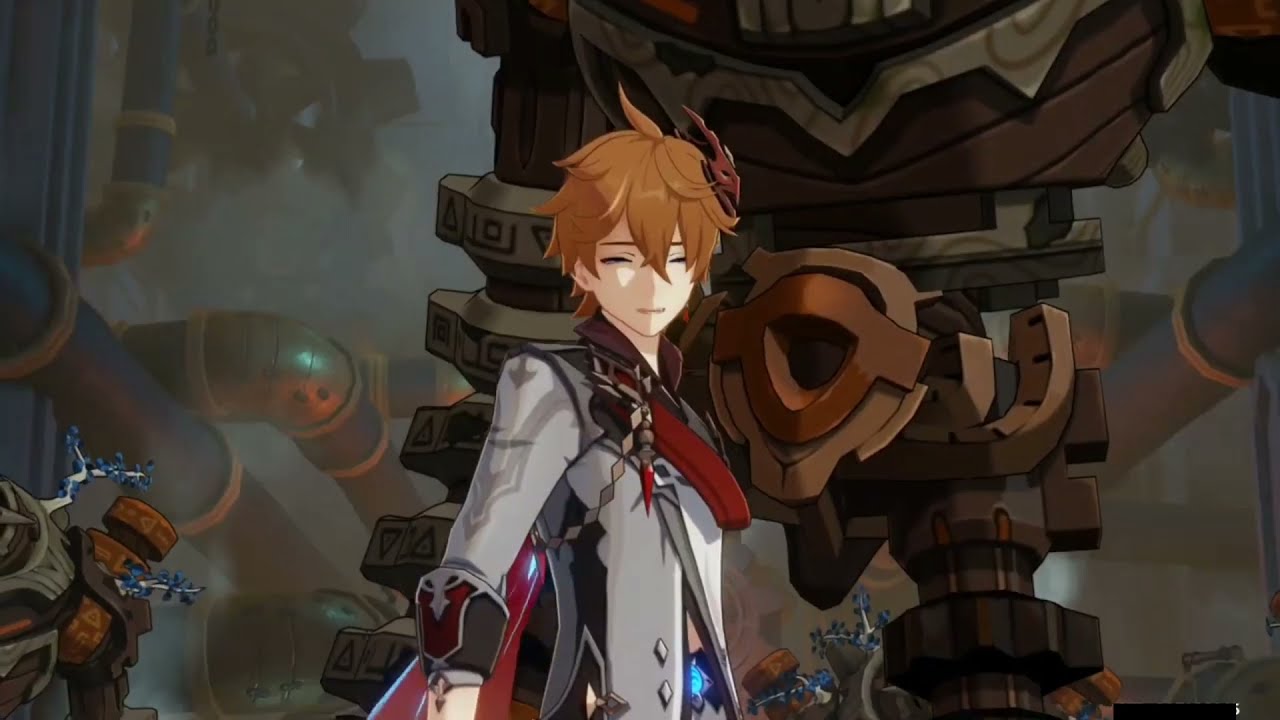The image, reminiscent of an anime or a video game screenshot, depicts a foggy, futuristic street scene filled with complex machinery. Central to the composition is a young character with unruly, light brown hair, styled in a spiky manner. Their expressive face, with squinting eyes, suggests a tranquil or content emotion. The character's gender remains ambiguous; however, they exude a warrior-like appearance, clad in a distinctive gray long-sleeved jacket featuring maroon or red and dark gray accents along the sleeves and collar. Below their jacket, a blue glow emanates from their waist. Behind them, a towering, humanoid robot constructed from various shades of brown material looms over their shoulder. To the left, massive navy blue pipes with gold-colored elbows and bindings contribute to the industrial vibe. Another smaller, robotic figure peeks out from the front left corner, adding to the scene's intricate mechanical setting.